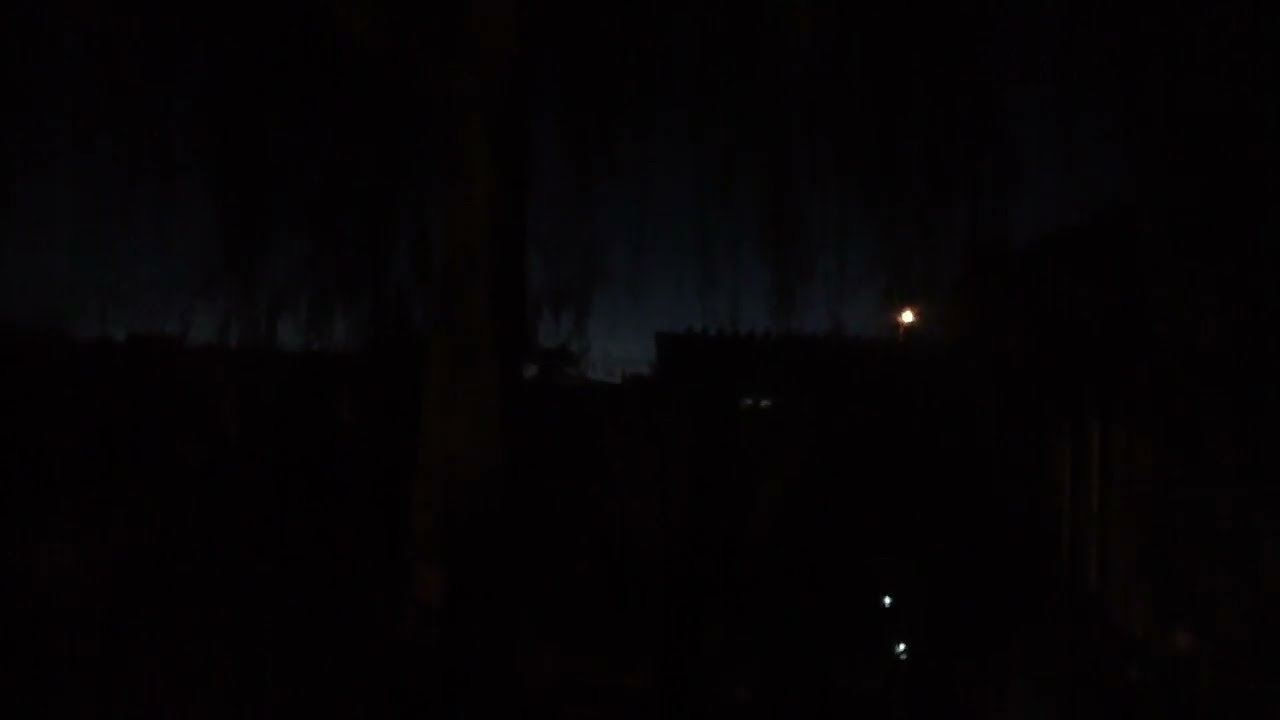The image depicts a predominantly dark, outdoor night scene with a faint, dark blue sky in the background. Along the horizon, a faint outline of buildings can be seen, highlighted by a streak of light running horizontally across the center. The most noticeable light is a warm, circular glow on top of a square building with some indistinct markings. Additionally, two small white lights are positioned one above the other on the center-right bottom. Delicate, low-hanging branches resembling those of a weeping willow tree are also slightly visible, casting black marks across the scene. There are possible tree silhouettes on the left side of the image, adding to the woodland ambiance. The entire scene, enveloped in darkness, is softly illuminated by these few sources of light, contributing to the serene yet mysterious atmosphere.